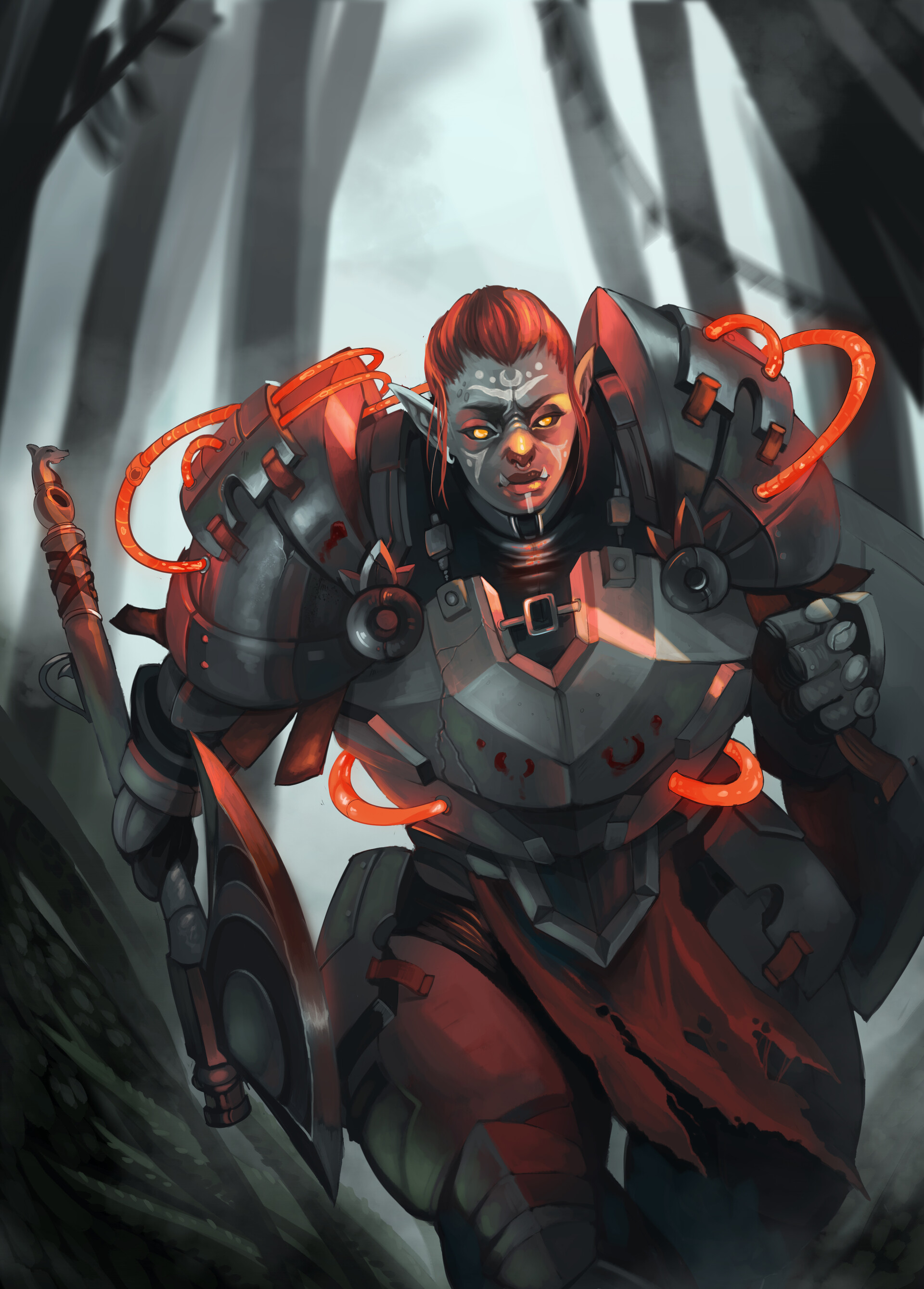An illustration in a sci-fi fantasy airbrush style, rendered in shades of black, gray, orange, and yellow, depicts a menacing warrior walking towards the viewer. This warrior features striking elf-like ears, vibrant long red hair with two bangs, and yellowish glowing eyes devoid of pupils. Their face is adorned with white or light gray face paint on the forehead and cheeks, possibly with piercings or jewelry on their lips. Clad in heavy, futuristic body armor with prominent shoulder pads connected by glowing orange tubes, the armor is a dominating silver. The chest piece has a V-shape design paired with a torn red loincloth, and they wield a large, sharp battle axe in their right hand. The background suggests a dense forest of towering, dark tree trunks against a gray sky, with steel-like beams complementing the eerie atmosphere.